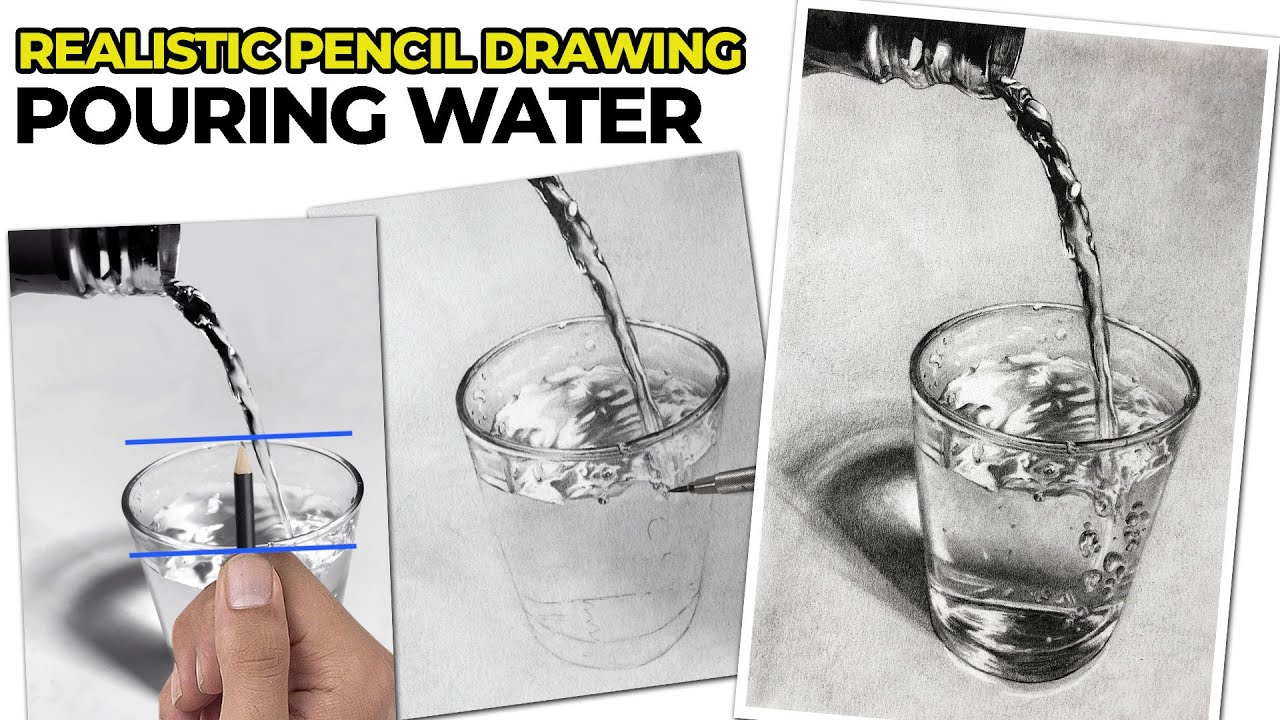The image displays a highly detailed realistic pencil drawing that serves as a video thumbnail, likely for a YouTube tutorial. At the top left, bold yellow sans-serif text in all caps reads "REALISTIC PENCIL DRAWING," outlined in black. Directly below it, in smaller, bold black sans-serif text, it says "POURING WATER." The image is divided into three main sections, illustrating various stages of a pencil drawing that depicts a bottle pouring water into a clear glass.

On the left side, an artist’s hand is superimposed over the drawing, holding a pencil with blue guidelines indicating the top and bottom edges of the glass. This demonstrates the scaling technique used in the drawing process. The middle image shows the partially completed drawing, focusing on the water being poured and detailing the top portion of the glass, with the bottom two-thirds remaining as rough sketches. The rightmost and largest image is the completed drawing, showcasing an extremely detailed and realistic depiction of water pouring into the glass, with visible bubbles and intricate shading. This final image highlights the shadows behind the glass and the realistic texture of the water.